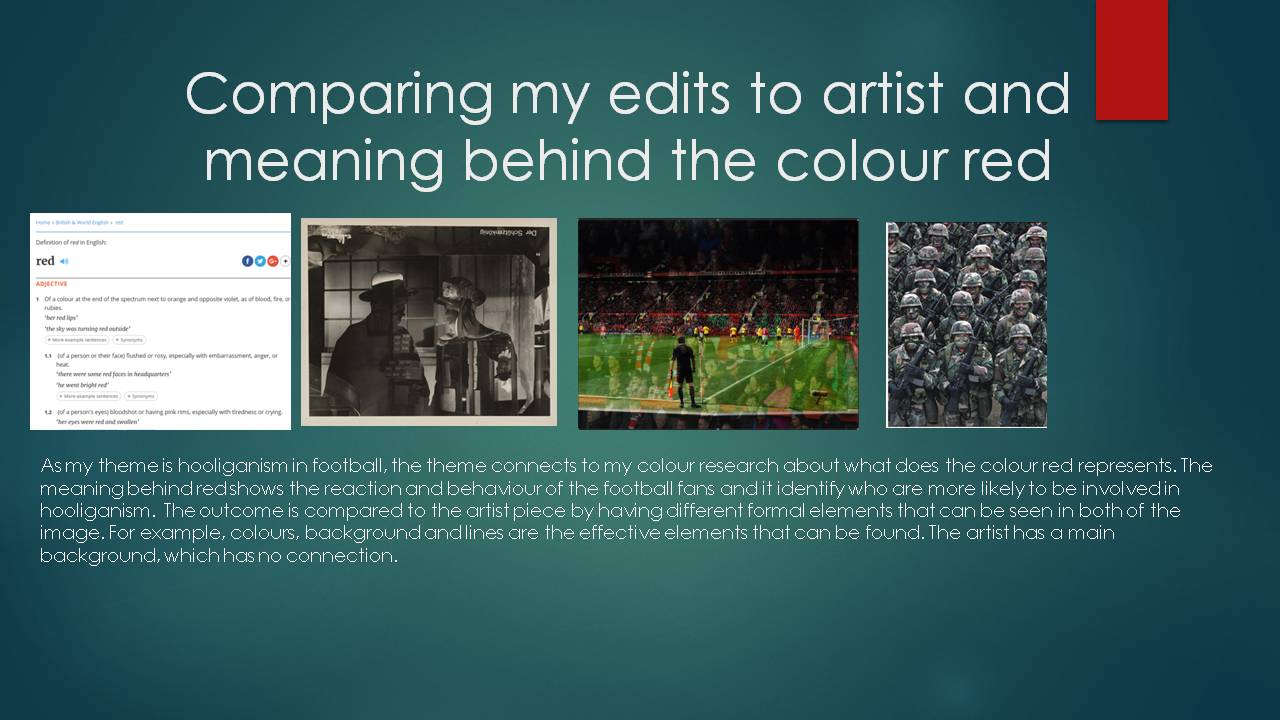The image is an advertisement with a wide rectangular format, featuring a gradient background that transitions from deep blue-green at the edges to a lighter greenish-blue towards the center. Centered at the top in large, basic white font, it reads: "Comparing My Edits to Artists and Meaning Behind the Color Red." A vertical red ribbon descends from the top right corner, aligning with the text. Below this heading, there are four distinct images arranged in a row:

1. The first image resembles a dictionary square, likely explaining the word "red."
2. The second image is a black-and-white photograph of two men facing each other.
3. The third image is a colored photo that appears to show a soccer field or green area with a person standing on it.
4. The fourth image is a monochrome photo, depicting soldiers standing in formation, possibly representing a military scene.

Underneath the images, in tiny white text, it elaborates on the theme: "As my theme is hooliganism in football, the theme connects to my color research about what does the color red represent. The meaning behind red shows the reaction and behavior of the football fans and identifies who are more likely to be involved in hooliganism. The outcome is compared to the artist's piece by highlighting different formal elements seen in both images. For example, colors, background, and lines are effective elements found in the artwork. The artist's main background is also noted for its lack of connection." The tiny white text appears to provide detailed information related to the research and interpretation of the images, linking them to artistic studies of color and behavior.